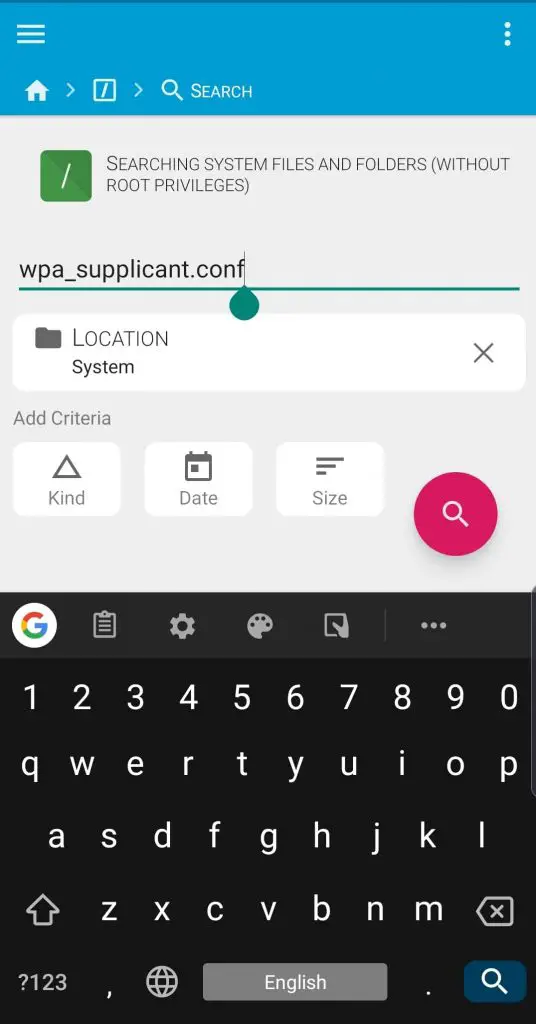This image depicts a screenshot taken from a smartphone. At the top of the screen, there is a tealish-blue rectangular bar containing essential status icons typical of a cellphone interface. On the far left of this bar, three horizontal lines are visible, while the far right displays three vertical dots aligned in a vertical position. 

Immediately below this bar, a row of navigation icons begins with a house icon, followed by arrows, and a white magnifying glass icon labeled "search". 

Further down, a green box stands out, containing the text "searching system files and folders" and an instruction in parentheses, "(without root privileges)". 

Moving downwards, there is a slight gap followed by the text "wpa_supplicant.conf" highlighted with a green underline. Adjacent to this, the word "LOCATION" appears in bold, all-capital black letters, and beneath it, the term "systems" is listed.

At the very bottom of the screen, a black keypad with white letters is seen, indicating a space for typing. The overall layout suggests an interface for searching and navigating system files on the smartphone.